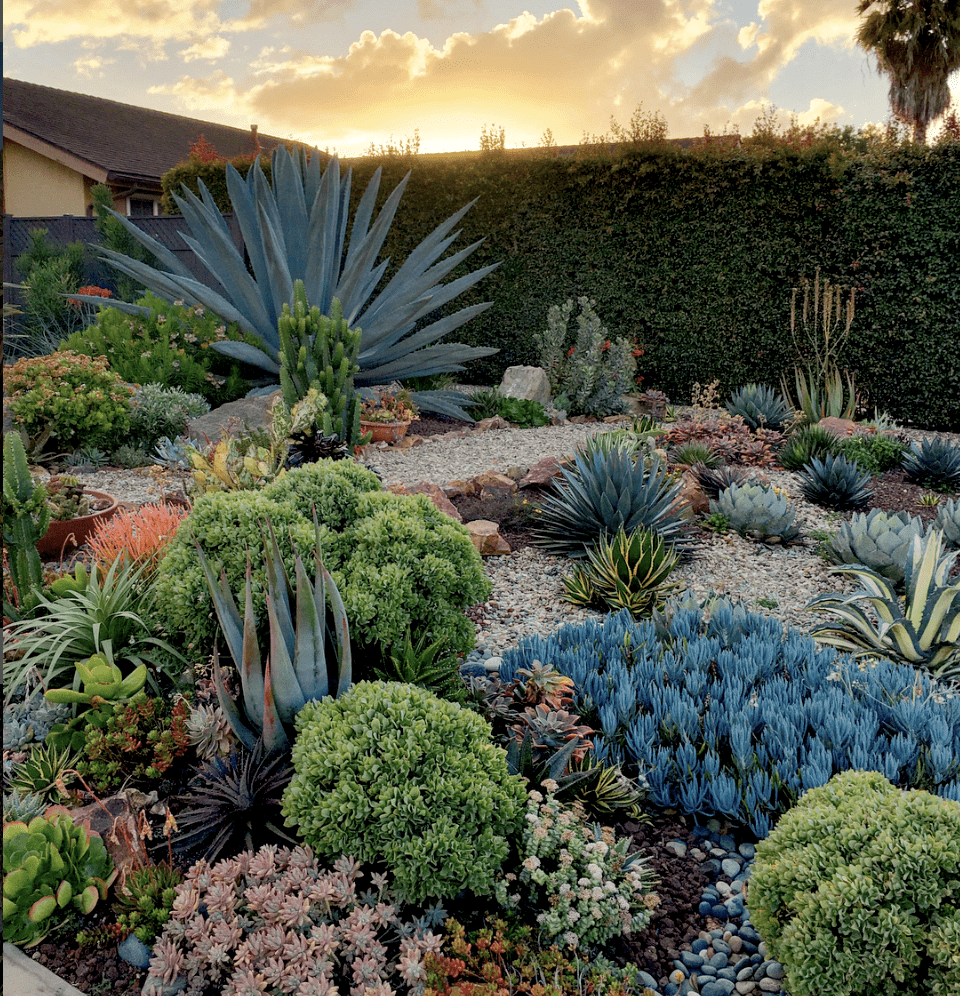The image showcases a vibrant and meticulously arranged garden dominated by a variety of cactus and succulent plants. These plants are diverse in shape and color, displaying an array of green hues—from light to dusty, deep green. Rounded cacti coexist with sharp-leaved succulents, while smaller bushes, including one reminiscent of a snake plant, add texture and depth. The garden is landscaped with stone pathways interspersed among the plants, creating a neat, clean appearance. There's a massive succulent on one side, standing out prominently. The backdrop features a green hedge, hinting at the garden's boundary, with a palm tree visible behind it. Beyond the hedge, a house with a brown roof is partially seen. Above it all, a blue sky filled with clouds, tinged with hints of orange and pink, creates a serene canopy over the garden.